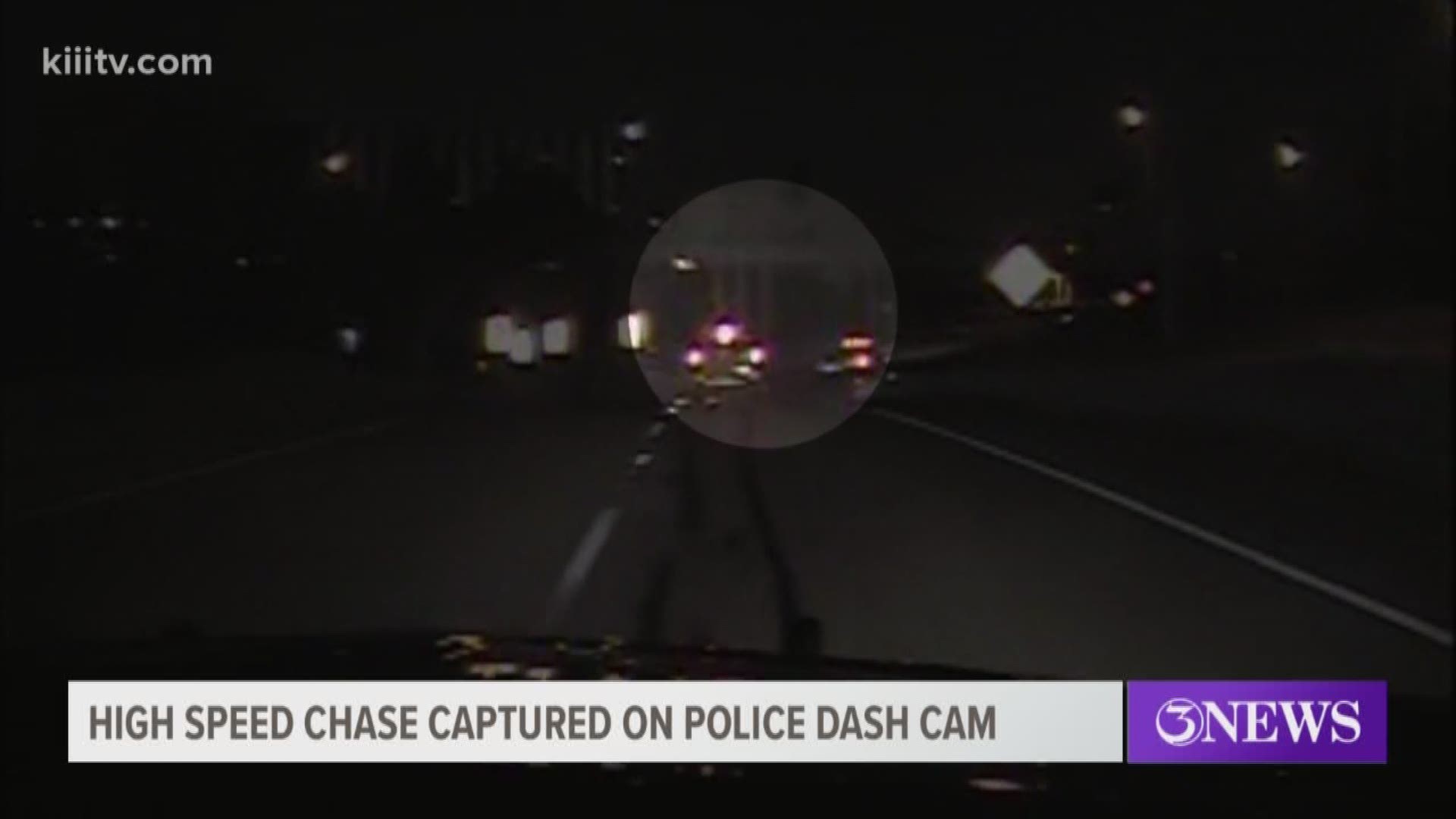This is a screenshot from a nighttime news broadcast, captured from a police dash cam video. In the top left corner, there is a white logo reading "kiiitv.com" against a black background. The image portrays a blurry, nighttime scene of a street or highway, illuminated by the headlights of the chasing police car and a few vehicles, likely pickups or SUVs, ahead. The center of the photo features a brightened circle highlighting the taillights of these cars, indicating a high-speed chase. At the bottom of the screenshot, a white rectangle chyron displays the text "High-Speed Chase Captured on Police Dash Cam" in black writing. Adjacent to this, on the far right, is a purple banner with "3 News" written in white. The overall scene, framed from the perspective of a police car's dashboard, shows the dashed white lines and solid boundaries of the two-lane road, with indistinct road signs reflecting the vehicle's headlights, emphasizing the pursuit in progress.